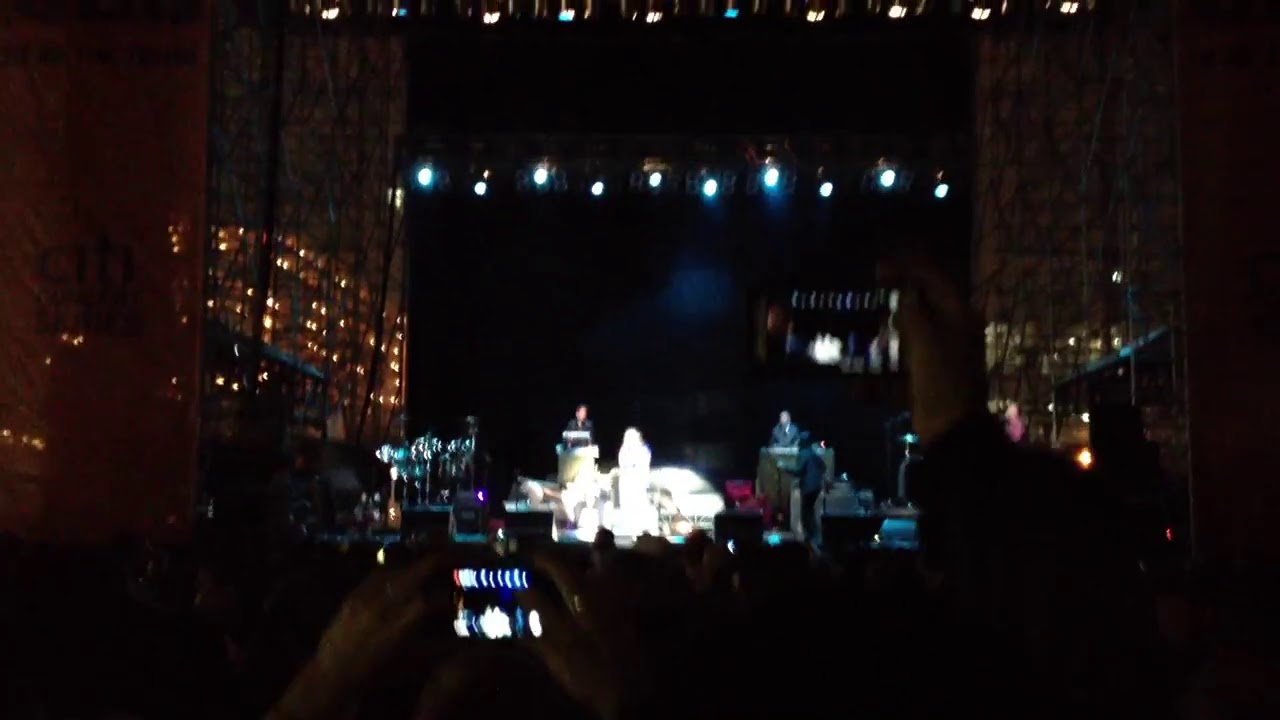The image captures a dimly lit concert hall, where a blurry but discernible stage is the focal point. Positioned in the middle left of the frame, someone in the audience holds up a smartphone or camera aimed at the stage. The stage is accented by overhead lights and a bright white spotlight that illuminates a central figure, presumably a singer. On either side of this central figure, there are additional performers, including a keyboard player. Reflective walls or curtains with lights add depth to the stage's left and right sides. Despite the image’s blurriness and low lighting, the stage's activities are partially visible, hinting at a lively performance that could be a concert or a theatrical play. A screen in the background also seems to display a live feed of the stage, enhancing the viewer's experience through the reflected and direct light.